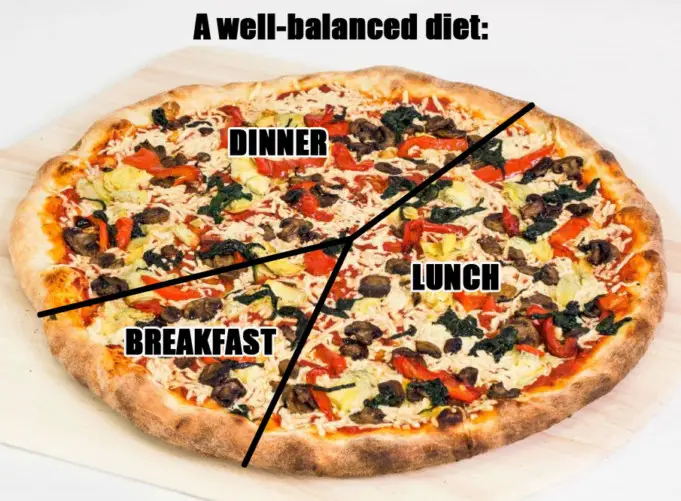This image features a well-balanced diet-themed pizza segmented into three distinct portions, similar to a pie chart. The segments are labeled with black text: the largest slice at the top reads 'Dinner', the medium-sized slice to the right reads 'Lunch', and the smallest slice at the bottom left reads 'Breakfast'. The pizza, adorned with various toppings such as mushrooms, peppers, tomatoes, and olives, sits prominently in the center of the image on a wooden pizza board. The scene is set against a clean white background, emphasizing the vibrant colors of the pizza and the thick crust beneath the melted cheese. Text at the top of the image, also in black, reads ‘A well-balanced diet’, tying the visual elements together.